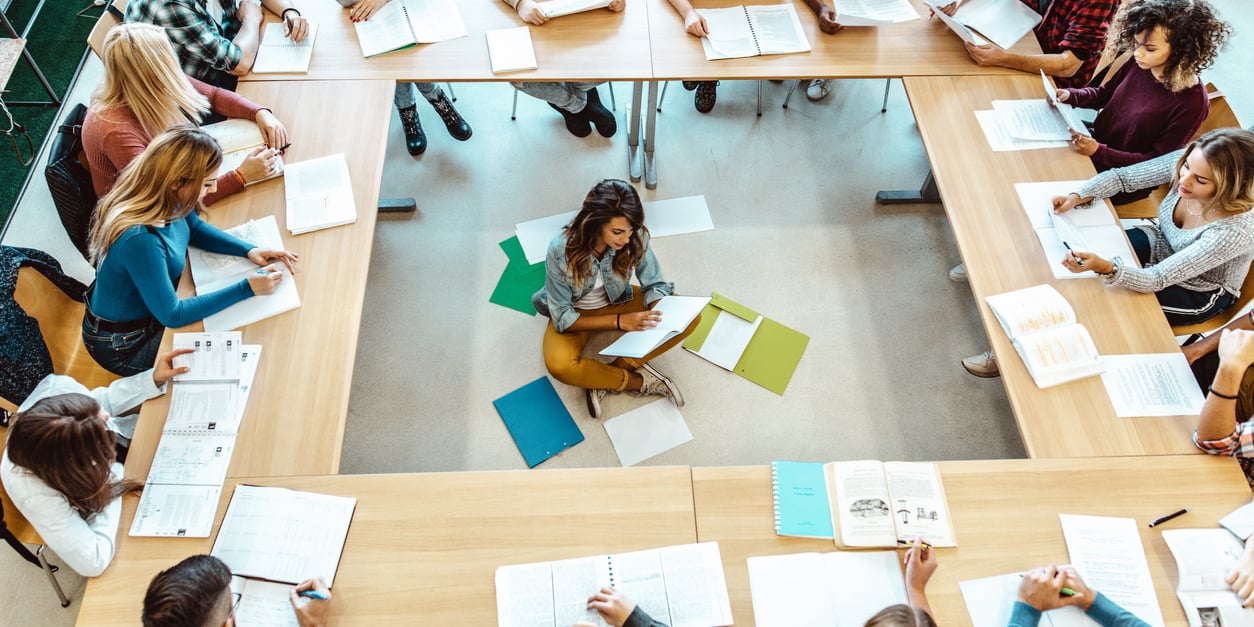The image is a horizontal rectangular photograph showcasing an unusual classroom setting from an overhead view. Several light tan rectangular tables are arranged to form a large square with an open space in the middle. Around the tables, numerous female students are seated, each with open notebooks, books, and writing utensils scattered in front of them. 

In the gray carpeted center of the square sits the teacher, a woman with long black hair, wearing a blue jean shirt and beige leggings. She is seated cross-legged on the floor, surrounded by various books, papers, and blue, green, and white folders. She holds an open book and appears to be reading or showing something to the students, who are attentively focused on her. The unconventional arrangement and the teacher's central position suggest a dynamic and interactive learning environment.